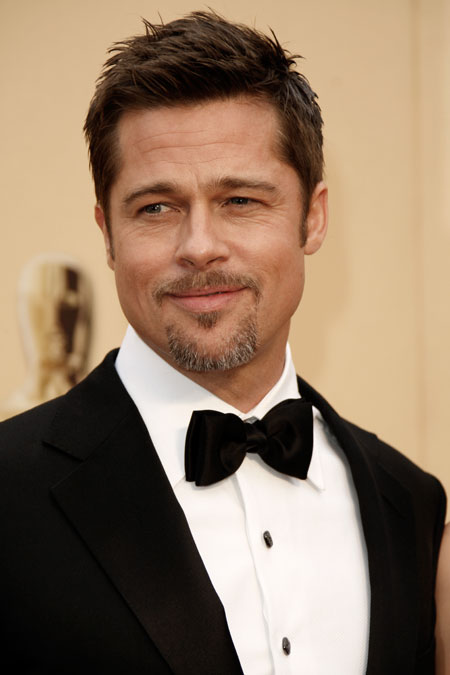The image features Brad Pitt, appearing as he did roughly a decade ago, dressed in a classic black tuxedo. He wears a black jacket, a black bow tie, and a white button-up shirt with white buttons. His short brown hair is styled into subtle spikes, and he sports a mustache and a salt-and-pepper goatee. Brad Pitt's complexion displays light-colored eyes and subtle wrinkles around his eyes and mouth, hinting at his age and adding character to his soft smile.

He's posing with his head slightly turned to the left, giving a gentle squint with his eyes and a smirk that reveals the warmth of his smile. The lighting in the photo casts more shadow on the left side of his face, while the right side is better illuminated. Standing against an off-white, almost beige, wall, there's a noticeable large gold oval towards the left side of the image that appears to resemble the face of an Academy Award, suggesting that this is a press photo taken at the Academy Awards. The background is slightly blurred to emphasize his presence in the image.